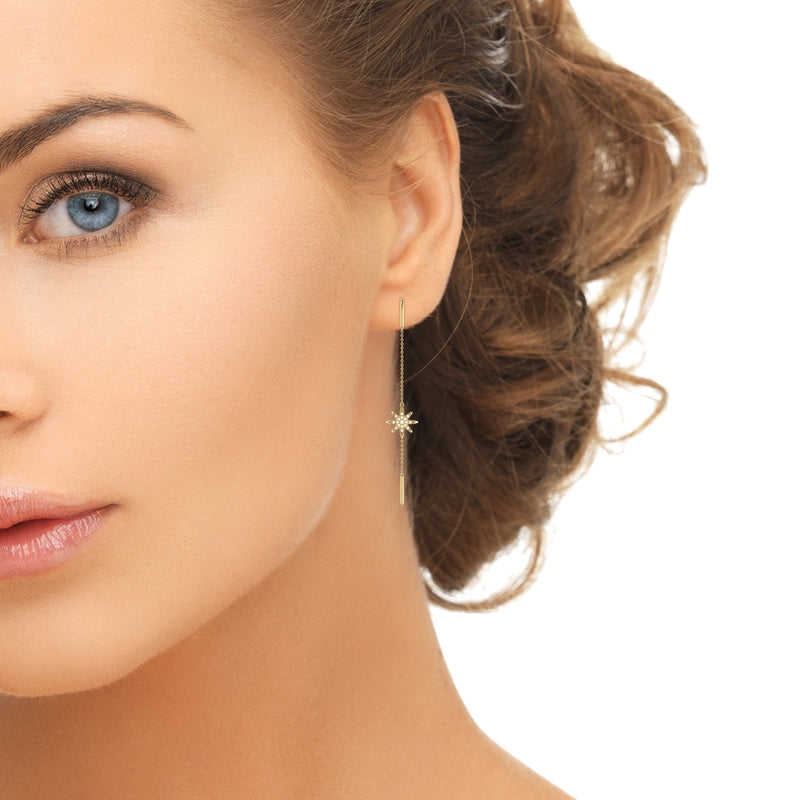This vertical, close-up portrait features the left side of a woman's face against a solid white background. The image highlights her striking blue eyes, light pink lipstick, and fair complexion, with minimal makeup that includes subtle mascara and brow definition. Her medium brown hair, slightly curled and pulled back, reveals a delicate gold dangling earring adorned with a sunburst design on an extremely thin gold chain. The earring, which measures around three inches long, accentuates her left ear, neck, and jawline. The soft, neutral expression on her partially visible face complements the overall simplicity and elegance of the composition.